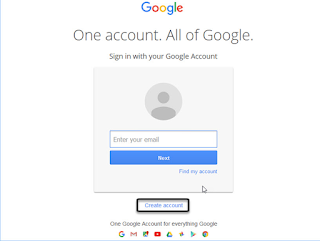This image is a screenshot of the Google account login page, set against a completely white background. A thin blue line runs vertically on the left and horizontally along the bottom of the image. At the top, the colorful "Google" logo is prominently displayed in blue, red, orange, blue, green, and red. Below this logo, grey text reads, "One account. All of Google," followed by another line that says, "Sign in with your Google Account."

In the center of the page, there is a very light gray box containing a circle with a generic silhouette representing a user’s profile picture, meant to be replaced by a personalized image upon account setup. Below this circle, a rectangular input box is labeled "Enter your email," and beneath it, another rectangular button labeled "Next." Below the "Next" button, there is a small arrow pointing to the "Find my account" link.

Towards the bottom of the light gray box, a smaller, heavily outlined rectangular button reads "Create account" in blue text. Underneath this box, another grey line of text states, "One Google Account for everything Google," accompanied by four small icons representing various Google services like Gmail, Google Maps, Google Photos, and the Google logo itself.